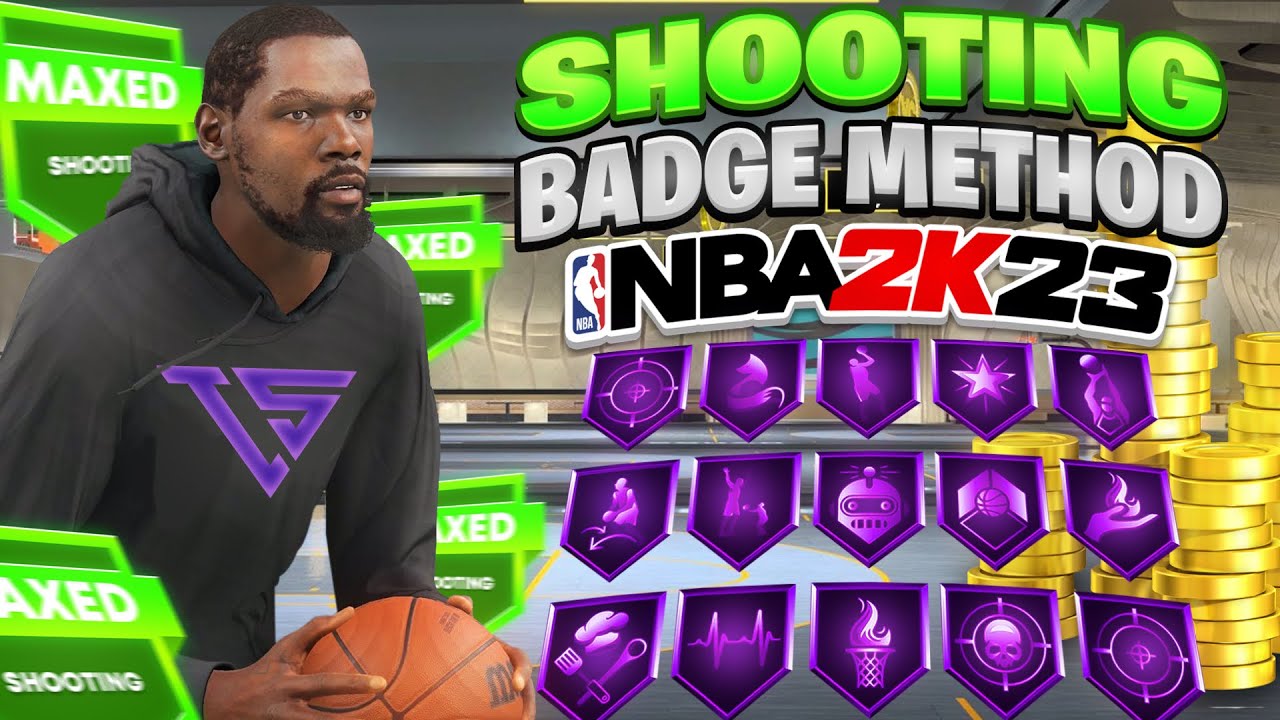The screenshot showcases an in-game scene from an NBA-themed video game, saturated with vibrant colors. Dominating the foreground is a basketball player, depicted as an African American individual, engaging in play. The screen prominently displays the phrase "Max Shoot" in eye-catching neon green, with the word "Shooting" in the same luminous green hue. A contrasting text, "Badge Method," appears in a white to gray gradient.

In the background, one can see a collection of small, shimmering coins. Additionally, the screen features a set of 15 purple shields, each adorned with distinct emblems, all gleaming with a glossy finish. These shields represent different badges, including four that are notably maximized.

The iconic NBA logo is visible, alongside the text "NBA," rendered in black with a white outline. Likewise, the game branding includes the text "2K" in red with a white outline and "2-3" in black with a white outline. Overall, this highly detailed screenshot captures the dynamic and immersive elements of the basketball video game.